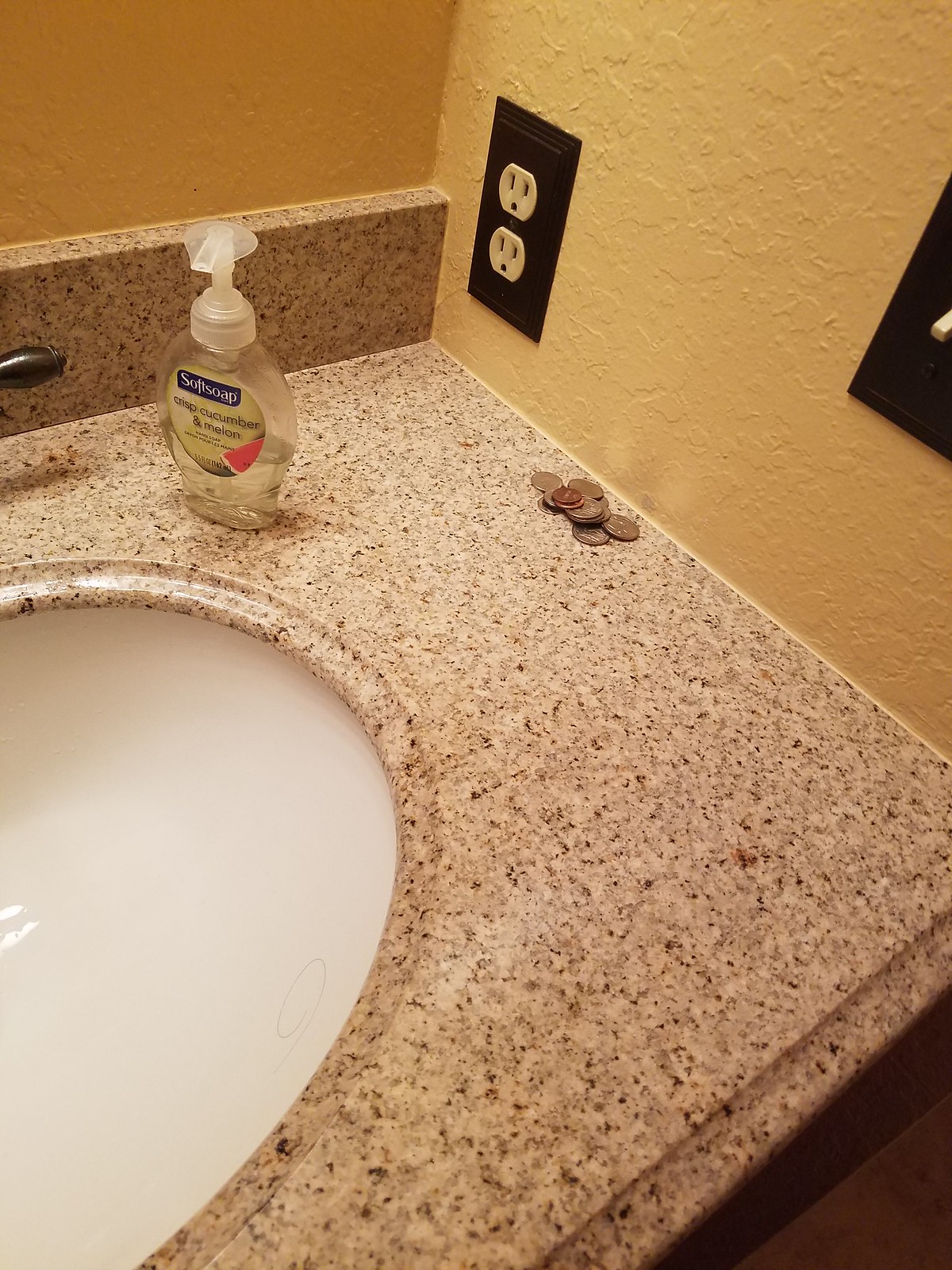In the background, the walls are painted a dark yellow color. A porcelain sink with a chrome handle is positioned under a smooth blue soap dispenser. The dispenser features a label indicating the scent as Crisp Cucumber and Melon, with text on the bottom right. The dispenser has a pump at the top, and the clear liquid soap is visible inside.

To the right of the sink, there's a pile of coins, primarily silver, with a lone penny on top. Above the coins is a black square, likely a switch plate, alongside a white light switch in the off position, yet the area is well-illuminated, suggesting the switch might control another light source.

The sink is clean except for a single strand of hair. The granite countertop below the sink has a mix of black, brown, and white speckles. This speckled pattern continues up a small backsplash lip at the back of the counter, which abuts the wall.

An electrical outlet is also visible on the wall, featuring two white sockets with three-prong holes (live, neutral, and ground). Reflections can be seen in the polished surface of the porcelain sink, adding to the overall brightness of the scene.